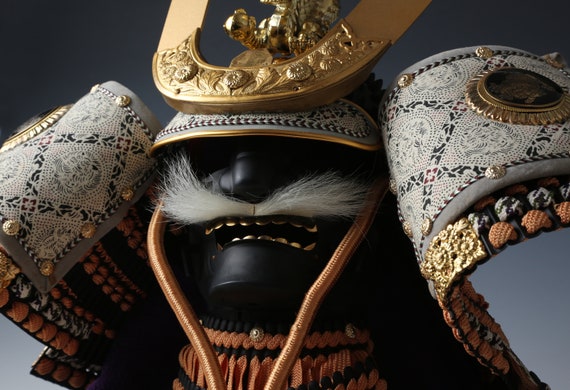The image depicts a highly ornate headpiece, resembling an artistic helmet or decorative armor, likely exhibited in a museum. The headpiece features an intricate design with prominent gold accents and embroidered fabric. At its center, there is a large, horseshoe-shaped piece with detailed floral carvings and tooled gold, reminiscent of the patterns found on tooled leather belts. The headpiece is adorned with a border of rope, adding to its elaborate appearance. It is mounted on a black mannequin or mask, which has a grimacing face with a white stringy mustache, yellowish rounded teeth, and no visible arms. This striking piece combines both elaborate craftsmanship and artistic elements, making it an intriguing artifact, hinting at cultural or ceremonial significance.